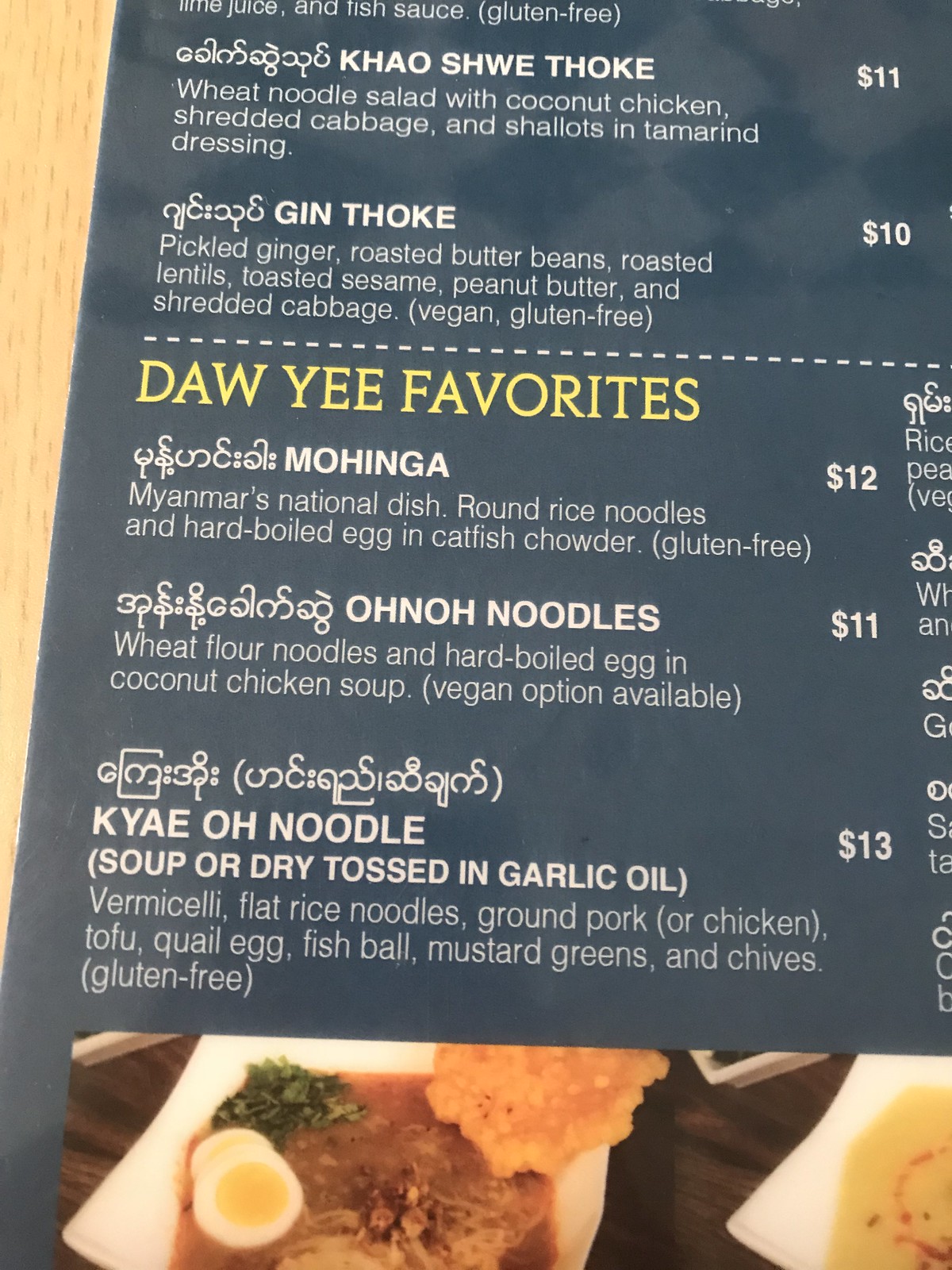This photograph captures a segment of a menu from a Myanmar cuisine restaurant. The menu features a sleek grey background with white text and section headings highlighted in bold yellow capital letters. At the bottom of the menu are vivid photographs that give a tantalizing glimpse of the restaurant's offerings. One of the displayed dishes consists of noodles served in a square bowl, accompanied by a rich sauce. Garnished with a halved boiled egg, vibrant green scallions, and a side of crispy fried dough, the dish appears both inviting and flavorful.

The menu prominently showcases a section titled "Do Yee Favourites" in yellow. Among the items listed under this section is 'Mohinga,' described as Myanmar's National Dish. The description elaborates that Mohinga consists of round rice noodles and a hard-boiled egg served in a savory catfish chowder, with a note indicating that it is gluten-free. The dish's name is also presented in Myanmar script, emphasizing its authenticity. Prices for each dish are clearly indicated next to their respective descriptions.